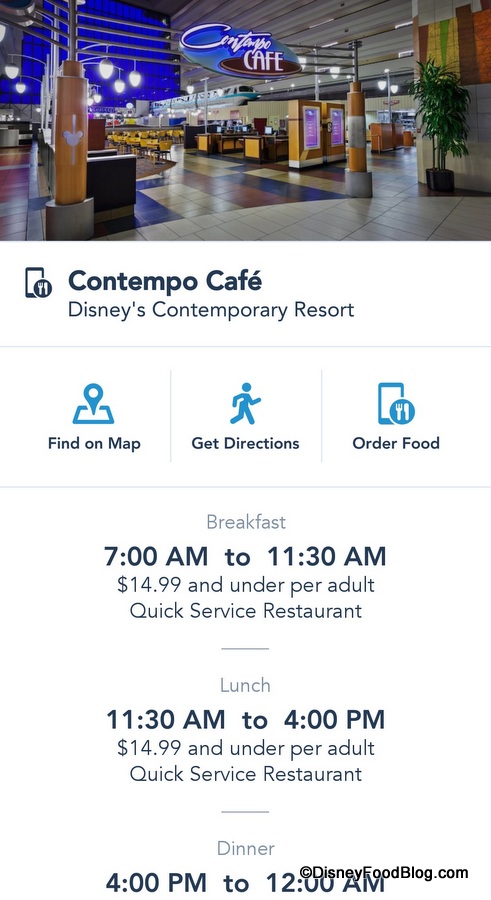This webpage features Contempo Cafe, located at Disney's Contemporary Resort. At the top, there's an image of the actual cafe which is currently empty, showcasing its spacious and modern design. The cafe has a lot of tables, a very open layout, and high ceilings. The decor includes royal blue accents in the background and bright, white lighting. Below the image, details include options to "find on the map," "get directions," and "order food."

The cafe offers quick service dining throughout the day:
- **Breakfast:** 7:00 a.m. to 11:30 a.m., priced at $14.99 and under per adult.
- **Lunch:** 11:30 a.m. to 4:00 p.m., also $14.99 and under per adult.
- **Dinner:** 4:00 p.m. to 12:00 a.m., with no specific pricing restrictions noted.

Further information can be found on DisneyFoodBlog.com.